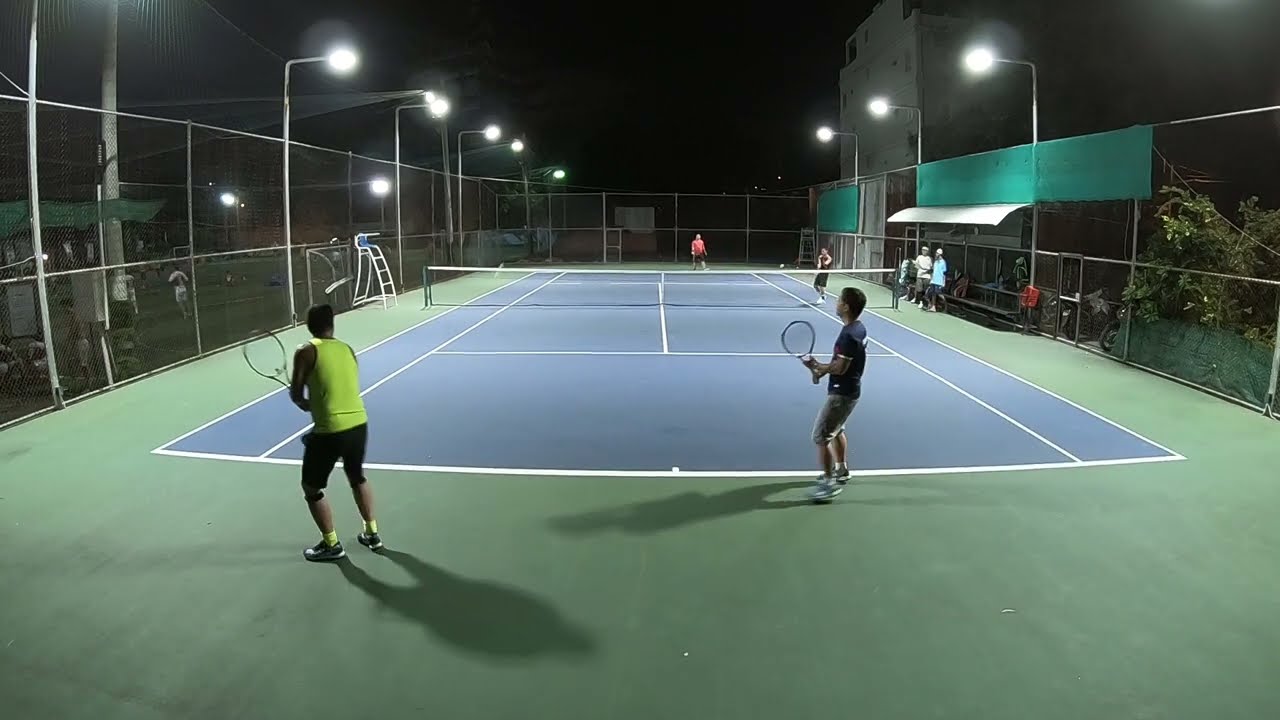In this nighttime scene, we view an outdoor tennis court illuminated by numerous light poles, casting a bright glow against the pitch-black sky. The blue court, marked with crisp white lines, is surrounded by a lighter green out-of-bounds area. Enclosing the entire scene is a tall, chain-link fence, approximately 10 to 15 feet high.

On the closer side of the court, two men are positioned: one donning a highlighter yellow shirt with black shorts and shoes, the other in a navy blue shirt with gray shorts and shoes. Each player grips a tennis racket, poised for action. Across the net on the opposite side stand two other players; one is dressed in red, and the other in black.

Adjacent to the court on the right, a white overhang shelters a bench area, where additional individuals observe the game. Some lean against the bench, while bicycles are parked nearby. In the background, outside the fenced perimeter, there are a few telephone poles and a distant building, contributing to the ambiance. The right side of the court also features areas of grass or greenery, alongside a visible tree, and additional courts are suggested beyond the left-side fence.